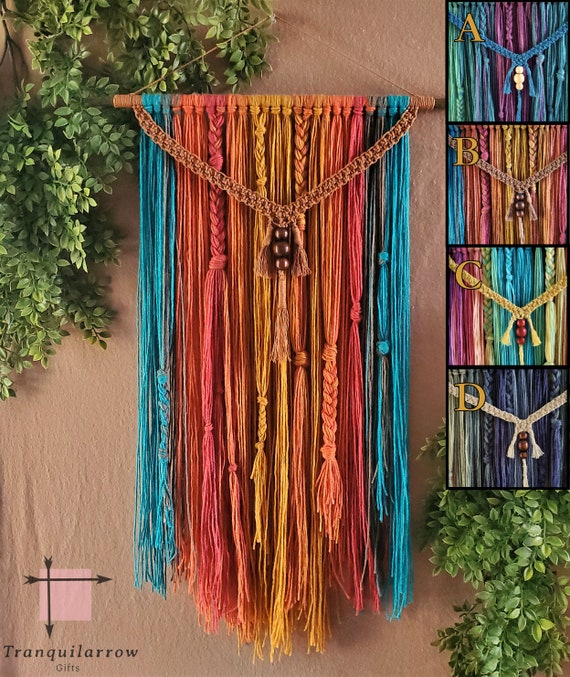This photograph captures a detailed and intricate macrame wall hanging crafted from yarn and cords in a harmonious palette of earth tones and vibrant colors, including teal, rose, coral, orange, gold, and yellow. The upper section of the macrame is meticulously tied around a rounded wooden rod, allowing the strands to cascade down. Some strands are intricately braided, creating dynamic patterns, while others are left to hang freely. Brown beads are incorporated into the design, adding an extra layer of texture and interest.

The wall hanging is displayed against a terracotta stucco wall, suggesting an outdoor setting adorned with surrounding greenery. This striking piece is labeled as a product by Tranquil Arrow Gifts, with options to customize colors to one's preference. Inset photographs to the left offer a glimpse of different color variations available for purchase, enhancing the versatility and appeal of the artwork. The entire presentation exudes a serene, bohemian aesthetic, with a nod to Native American craftsmanship.